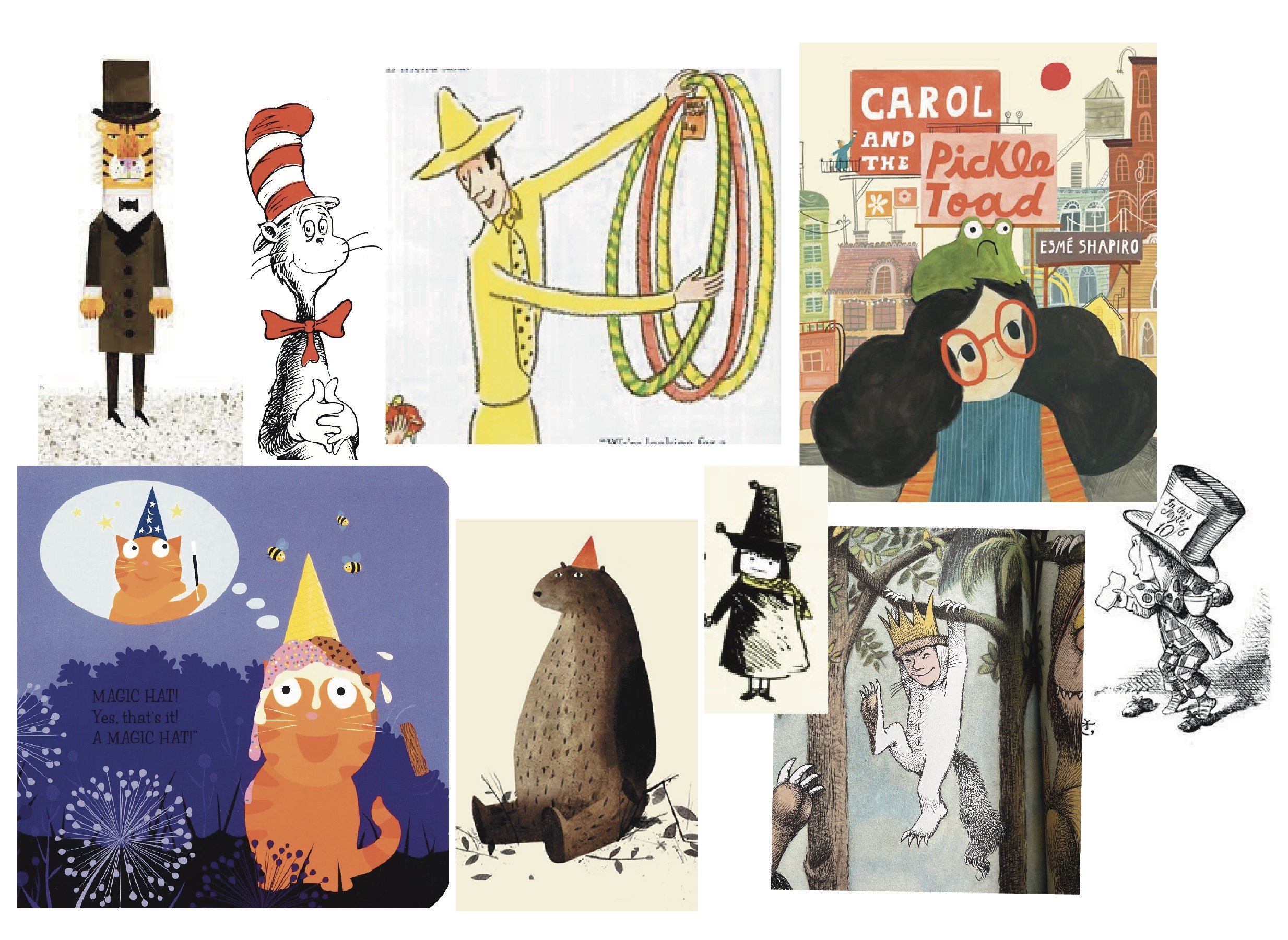The image is a composite artwork featuring a series of cartoonish illustrations, each in its own frame, and appears to be a collection of covers or illustrations from children's books. In the upper left corner, there's a depiction of a tiger dressed in a large black top hat, black coat, and a black bow tie. Below this, an orange cat wearing a cone on its head, surrounded by bees, is imagining itself in a wizard hat. Adjacent to the tiger, there is a classic "Cat in the Hat" illustration with the cat sporting a tall white and red striped hat and a red bow tie. To the right, a Mexican man stands dressed entirely in yellow, holding a collection of ropes. Directly next to him, a little girl with big red glasses and large black hair is illustrated with a toad on her head under the title "Carol and the Pickle Toad." The lower part of the composition includes a whimsical scene of a bear wearing a red hat sitting in a forest and an assortment of other black-and-white doodles, such as a witch, a boy in a white onesie and crown swinging from a branch, and a man with a top hat. This eclectic and colorful array of characters and scenes brings a playful, storybook-like atmosphere to the entire image.